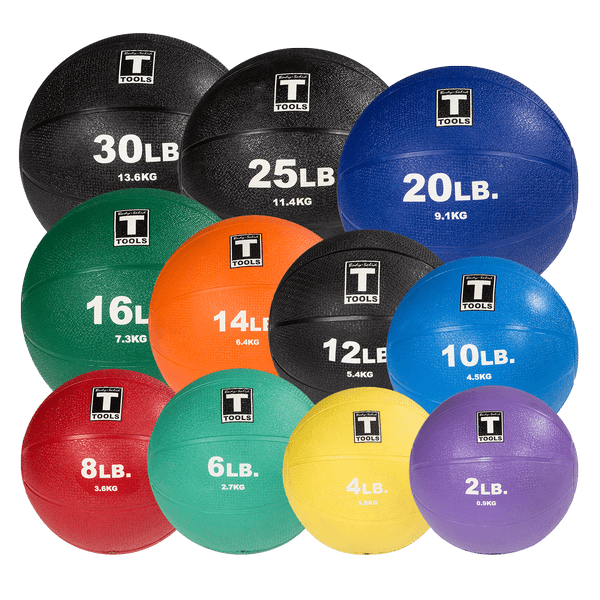This photograph displays an array of weighted exercise balls arranged on a white background, showcasing an assortment of vibrant colors and labels detailing their respective weights. Starting from the bottom right and ascending to the top left, the lightest ball is a 2-pound violet ball, followed by a 4-pound yellow ball, a 6-pound light green ball, an 8-pound red ball, a 10-pound light blue ball, a 12-pound black ball, a 14-pound orange ball, a 16-pound dark green ball, a 20-pound dark blue ball, a 25-pound black ball, and finally, a 30-pound black ball. Each ball features a black square logo with a large white "T" above the word "TOOLS" and includes the weight in both pounds and kilograms, such as "8 LB" with "3.6 kg" beneath. The arrangement starts with four balls on the bottom row, four in the center, and three at the top. The balls' colors—purple, yellow, light green, red, dark green, orange, light blue, dark blue, and three black—add visual variety, emphasizing the progressive weight increase from lightest to heaviest.